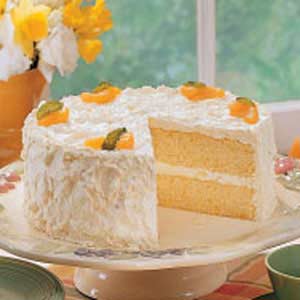The image features a vertical, indoor photograph of a two-layer, yellow cake with white frosting, perched on a white ceramic platter with a low stand, resembling an upside-down bowl. The cake, adorned with orange slices on top, has a V-shaped piece missing, revealing its yellow interior. The platter is embellished with colorful decorations, possibly red and purple flowers with green leaves, encircling the cake. A small, light green cup is positioned in the lower right corner, while a white bowl with a dark interior rim sits on the other side. This setup rests on a countertop, covered with a red, orange, and brown plaid tablecloth. In the background, a window reveals lush green vegetation outside, implying an overcast day with diffused ambient light. The window is framed with white wood trim, and positioned in the upper left corner is an orange planter with vibrant white and yellow flowers, enhancing the cozy, indoor setting.